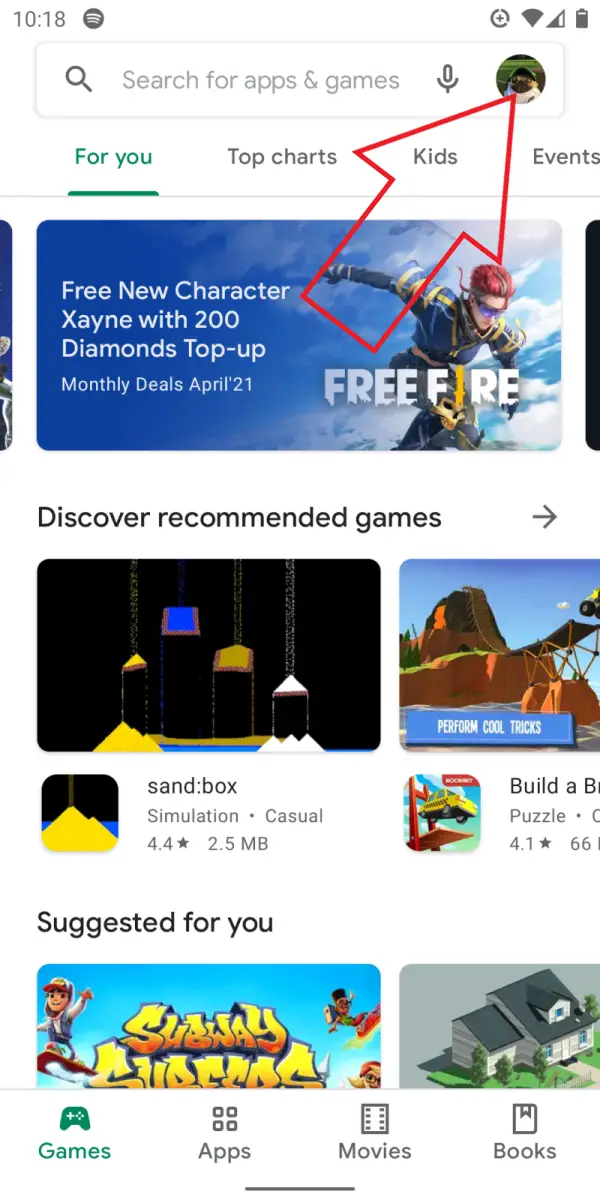This is a screenshot from the Google Play Store, captured on a mobile phone with a white background. The upper left and right corners display phone status information in gray: on the left, the time reads 10:18 and there is a Spotify logo; on the right, there are icons for a plus sign, Wi-Fi, mobile signal strength, and battery level. 

Just below these icons, there's a search field featuring a magnifying glass icon on the left, a text prompt saying "Search for apps & games" in gray font in the middle, and a microphone icon on the right. At the far right edge is a small profile picture associated with the user's Google account, highlighted by a photoshopped giant red arrow pointing at it.

Directly under the search field is a menu bar with categories 'For you,' 'Top charts,' 'Kids,' and 'Events,' with 'For you' currently selected. Beneath this menu is a rectangular advertisement for the game Free Fire. The advertisement features a background resembling a blue sky and shows a video game character dressed in cyberpunk gear walking towards the right, wearing sunglasses. In white font on the left side of the ad, it reads: "Free new character Zane with 200 diamonds, top up."